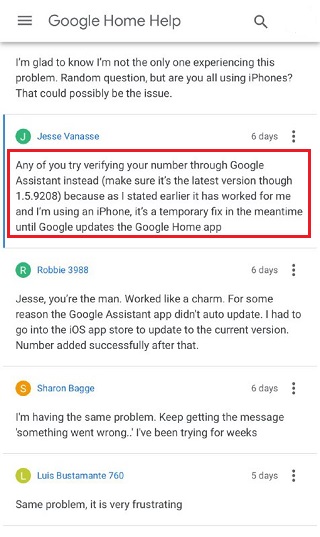Screenshot of a Google Home Help forum showing various user interactions. At the top, there is a navigation menu icon represented by three horizontal lines, followed by the title "Google Home Help" to the right. Next to the title is a magnifying glass icon, all sitting above a light gray colored line. Below this, in black text, a user comments, "I'm glad to know I'm not the only one experiencing this problem. Random question but are you all using phones or iPhones? That could possibly be the issue."

Further down, another light gray line separates the previous comment from a user identifier featuring a green circle with the initial "J" inside, followed by "Jesse Vanassie, 6 days ago." Below this, an outlined paragraph highlighted with a red rectangle contains the user comment: "Any of you try verifying your number through Google Assistant instead? (Make sure it's the latest version though 1.59208). Because as I stated earlier, it has worked for me and I'm using an iPhone. It's a temporary fix in the meantime until Google updates the Google Home app."

At the bottom of the screenshot, there's another user identifier with a green circle containing an "R" and the name "Robbie 3988" in blue text. This user replies, "Jesse, you're the man! Worked like a charm."